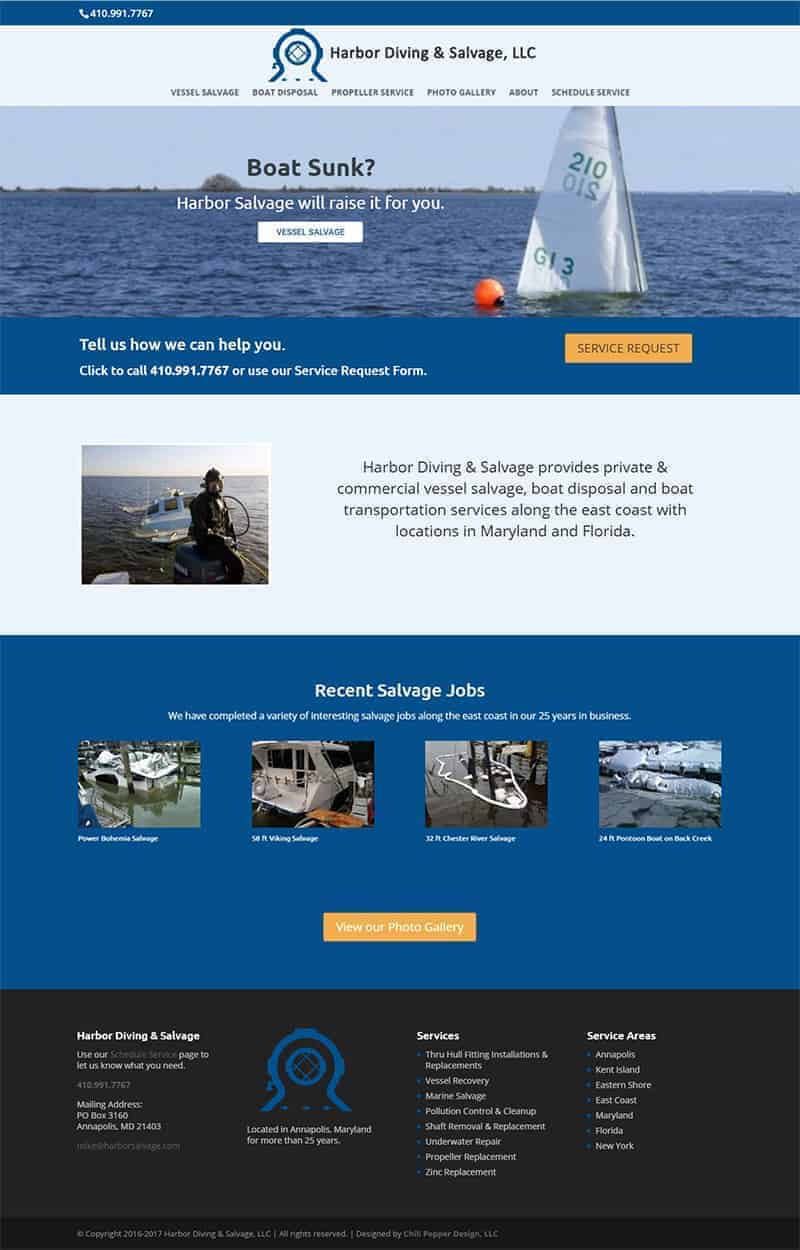Here is a cleaned-up and detailed caption for the described image:

"A screenshot of the Harbor Diving and Salvage LLC website. At the top, the site name is prominently displayed. Below it, there are six small, black-text categories. The central section features a sailboat on a serene blue body of water beneath a light blue sky, with the text 'Boat sunk? Harbor Salvage will raise it for you' overlaying the scene. Below this, a white rectangle with an interactive option is presented. Adjacent is a dark blue section extending side-to-side, containing white text and a yellow rectangle also with an option. Farther down, there's an image depicting someone on the water accompanied by a couple of sentences in black text against a light blue background. Next, a blue section showcases the heading 'Recent Salvage Jobs' with four images lined from left to right, each captioned with very small white text naming the job. Lastly, a light orange rectangle with white writing is visible before reaching the bottom of the website, which features a black background. It includes a mirrored black-and-blue design in the center flanked by very small text on both sides."